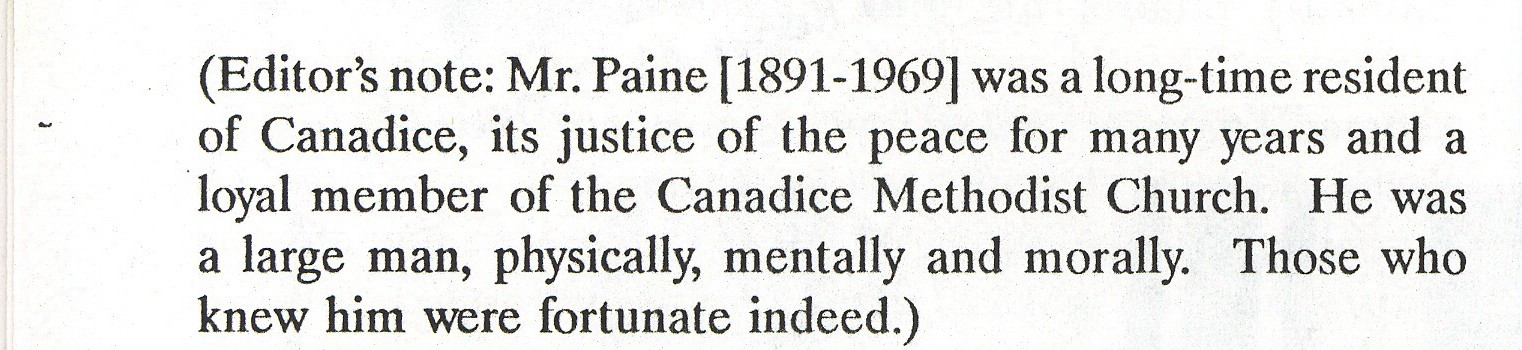The image depicts a simple white poster with black lettering, featuring an editor's note clearly framed within parentheses. The text reads, "Editor’s Note: Mr. Payne (1891-1969) was a longtime resident of Canada’s Cannadice, serving as its Justice of the Peace for many years and as a loyal member of the Cannadice Methodist Church. He was a large man, physically, mentally, and morally. Those who knew him were fortunate indeed." The entire note appears to add context to a larger piece, resembling an excerpt from a book or a webpage with no additional borders, trims, or colors, presented in a straightforward paragraph format without indentation.